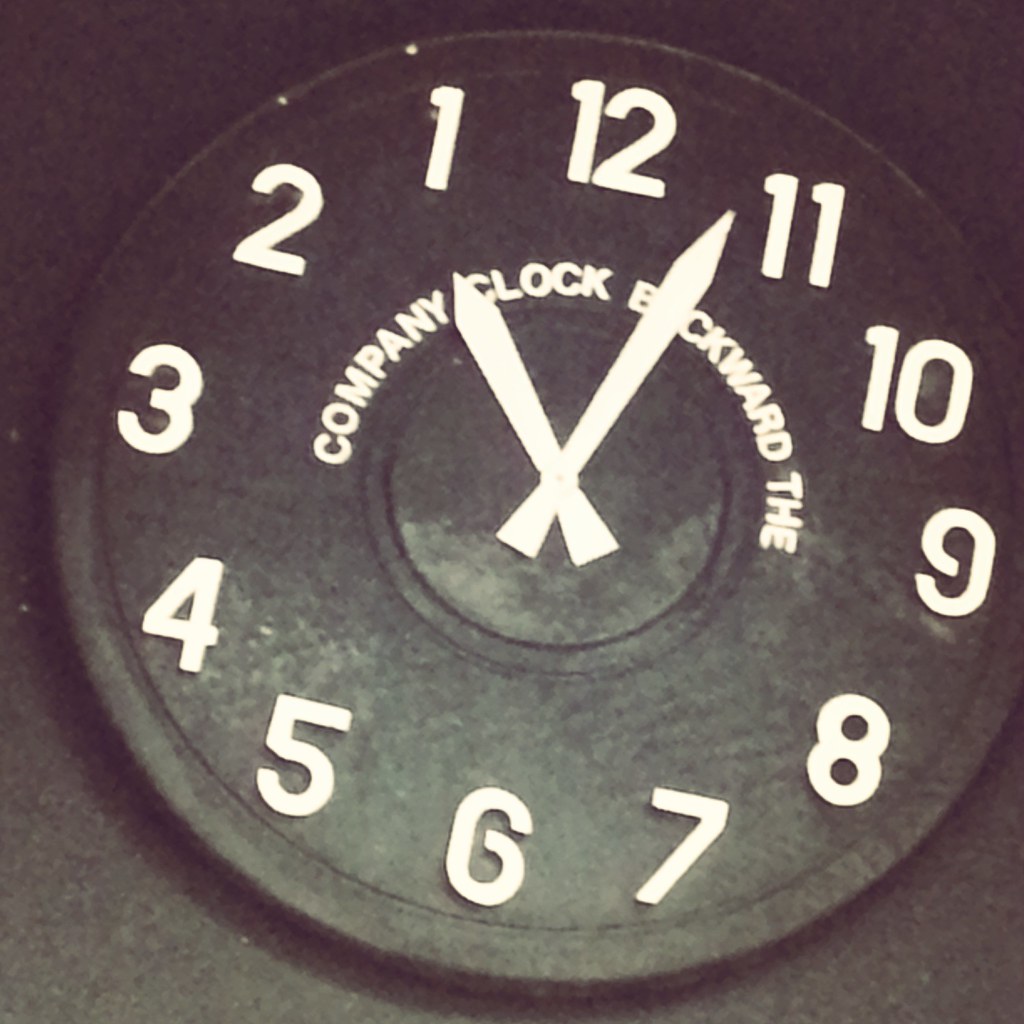This photograph showcases a unique clock hanging on a black wall, with both the clock and the wall sharing a similar texture that creates a seamless visual effect. The clock face itself is black with white numbering and hands that provide a stark contrast. Interestingly, the numbers on the clock are arranged in a reverse sequence, starting from 12 and descending counter-clockwise through 11, 10, 9, and so forth. The white hands of the clock indicate a time of approximately 2:50, with the smaller hour hand pointing slightly past 2 and the larger minute hand positioned between 11 and 12. Adding to the quirkiness, a playful touch is evident in the clock's design: the company's name and logo are written backwards along the curve of the clock face, aligning with the overall theme of reversed elements.